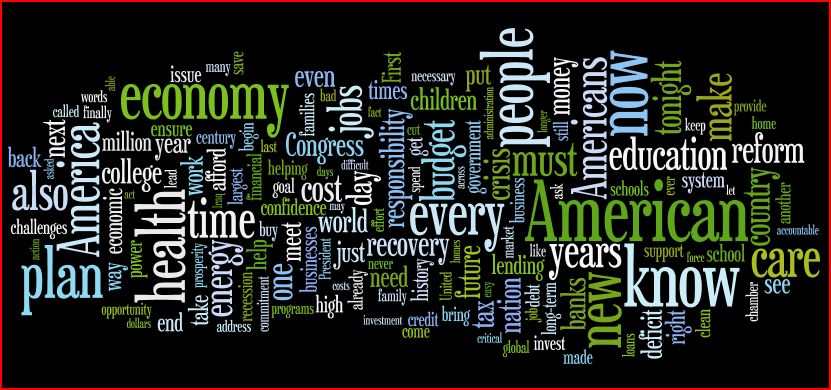The image, rendered in a print style, features a black background with a thin red border along the edges. Scattered across this canvas are numerous words in varying shades of blue, green, and white, all predominantly lowercase. The words, devoid of any specific arrangement, represent various themes and concepts. Key terms include "economy," "recovery," "jobs," "college," "health," "education," "plan," and "reform." Additional words, such as "challenges," "family," "energy," "commitment," "recession," "confidence," "Congress," and "opportunity," intermingle in a dynamic pattern. The diverse color palette and haphazard placement of the words create a visually engaging and textually dense presentation, emphasizing themes pertinent to national and economic discourse.